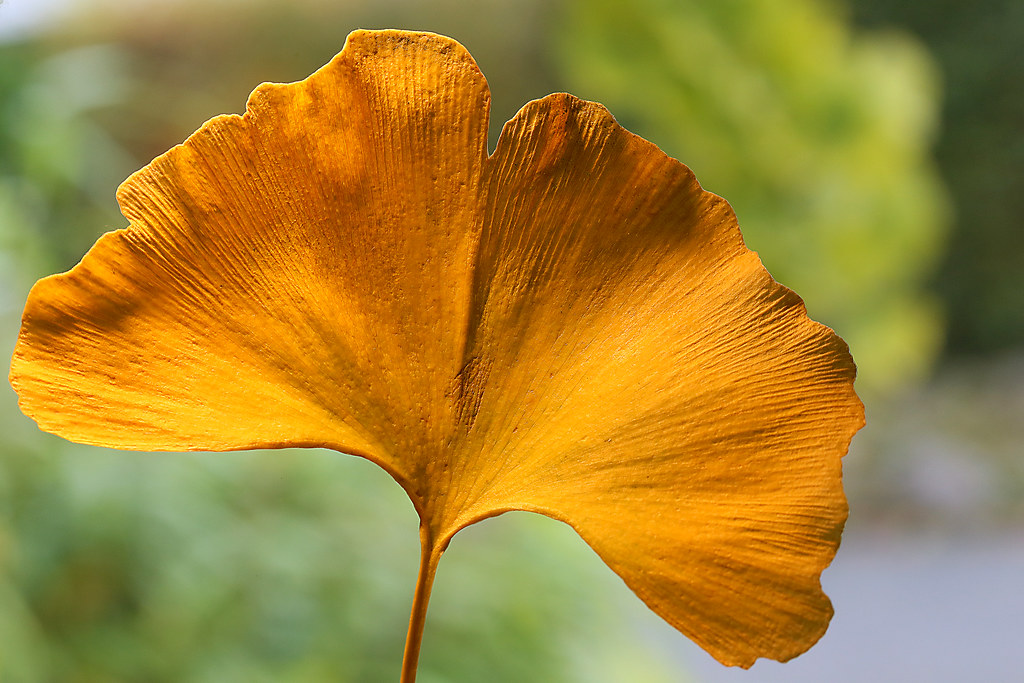A stunning, highly detailed close-up photograph captures the intricate beauty of what appears to be a leaf, though it evokes the delicate appearance of a flower petal. This broad yellow-to-amber leaf exhibits a beautifully irregular, almost scalloped edge and is shaped somewhat like a clover, with two large lobes fanning out to the sides and meeting at a slender stem. The leaf's textured striations run prominently from tip to base, giving it a nearly symmetrical, yet naturally unique look. The leaf is imbued with shades of yellow, amber, and orange, with the sunlight casting compelling shadows and highlights across its surface. The background, rendered in a blurred mosaic of green hues, suggests a natural outdoor setting, perhaps among trees or bushes, ensuring that the viewer's focus remains entirely on the finely detailed foreground. The photograph itself, masterfully composed, draws the eye to the leaf's striking colors and textures, featuring a sharp foreground that contrasts beautifully with the softly obscured, verdant background.